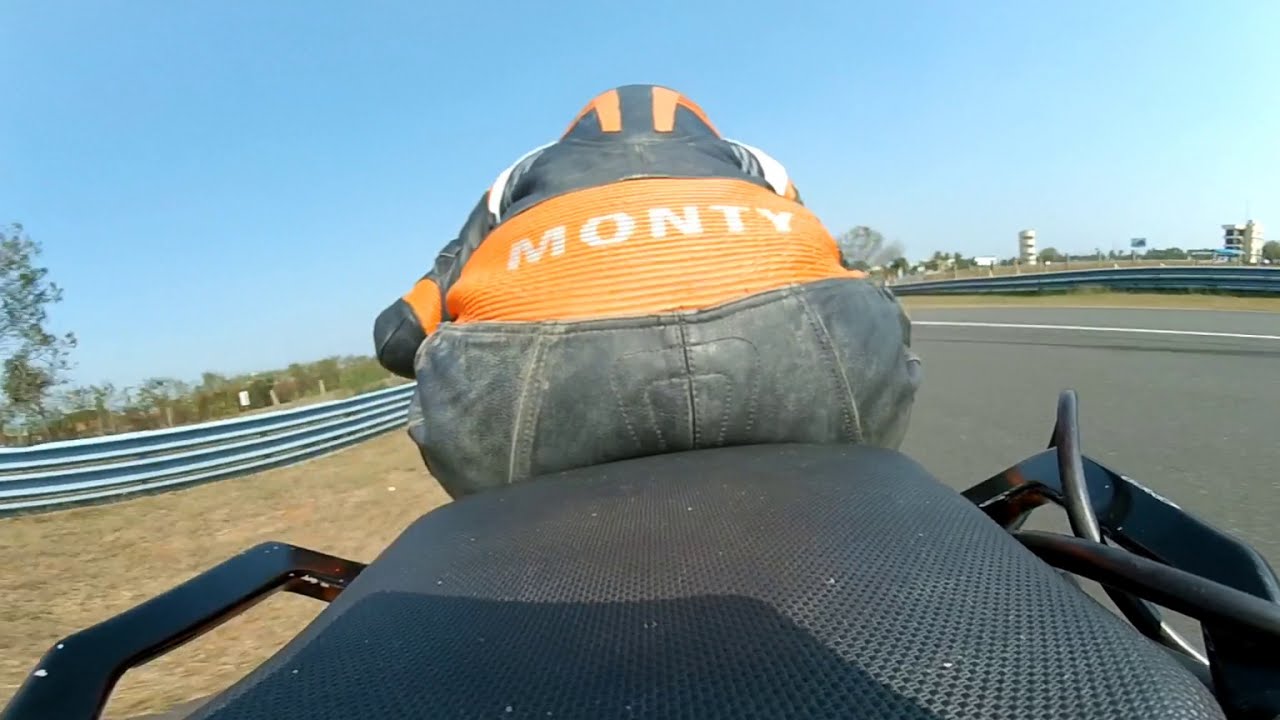In this image, we're looking at the back of a person bent over on a motorcycle from the perspective of the seat. The individual is clad in black leather pants, a black motorcycle jacket, and a black helmet with orange stripes. An orange band around their waist prominently features the word "Monty" in white capital letters. The black seat they're riding on has noticeable perforations and a visible cable around the right handle. The scene is set on a clear day with a vibrant blue sky. The motorcycle is traveling down a highway, flanked by guardrails on both sides. On the left edge of the image, there's a tree, and small buildings are visible on the right. The person and the "Monty" band are positioned centrally, making them the image's focal point.